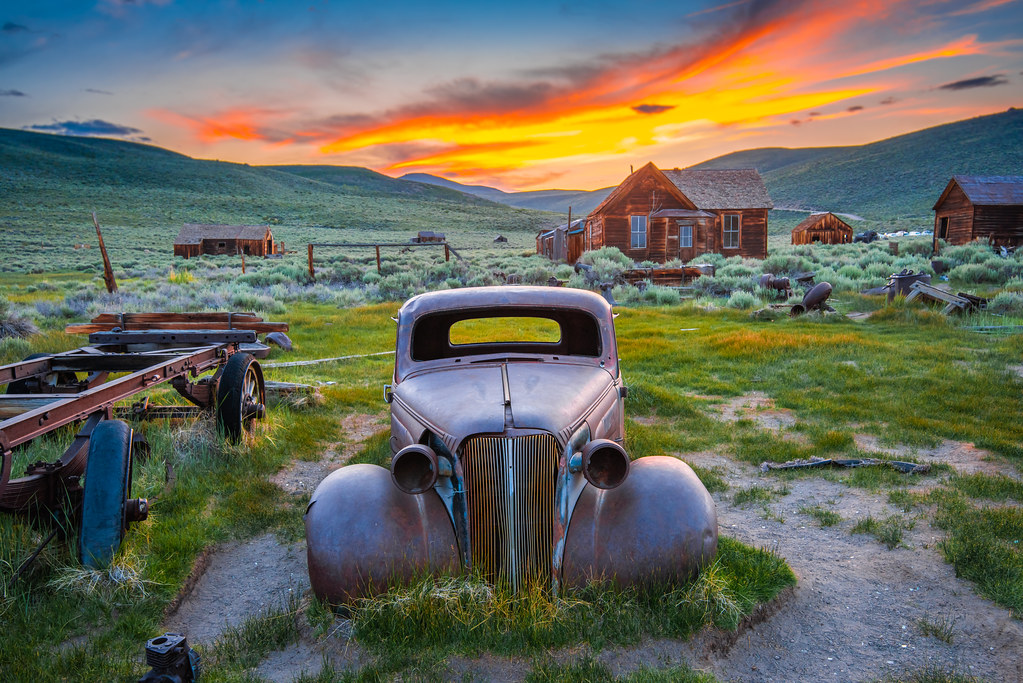In this vibrant, detailed image, the foreground prominently features the rusting front half of an old-fashioned vehicle from the 1940s or 50s, with its headlights facing directly at the viewer. The setting appears to be a vast, grassy farm or field, with patches of dirt interspersed throughout. On the left side of the image, there is a piece of farming equipment, adding to the rural ambiance. The background reveals several wooden structures that resemble log cabins or barns, their details blurred due to distance. The sky is a stunning mix of bright orange and yellow hues, suggesting either sunrise or sunset, and it casts a warm glow over the entire scene. This picturesque moment, whether captured in a photograph or a digital artwork, magnificently blends natural beauty with elements of rustic decay.